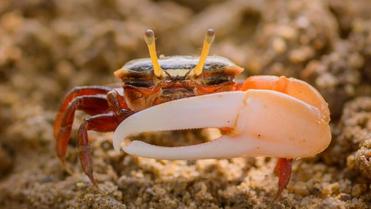This image captures a small, vividly detailed crab standing on coarse, brownish sand speckled with black grains. The crab's body is a striking blend of colors: its top shell is black, transitioning to reddish-brown towards the legs, which are also red. The crab's most prominent feature is its single, large claw on the right side. This claw exhibits a gradient of colors, starting whitish at the tip, turning pink near the elbow, and finally merging into an orange-red closer to the body. Its eyes, perched on extended yellow stalks, have black tips, giving it a distinctive, almost alien appearance. The crab's semi-translucent shell allows light to filter through, adding an ethereal quality to its form. Despite its small size, the creature's dynamic pose and sharp, pointy legs make it look ready for action, as if it’s posing for the photograph in a wildlife documentary setting.